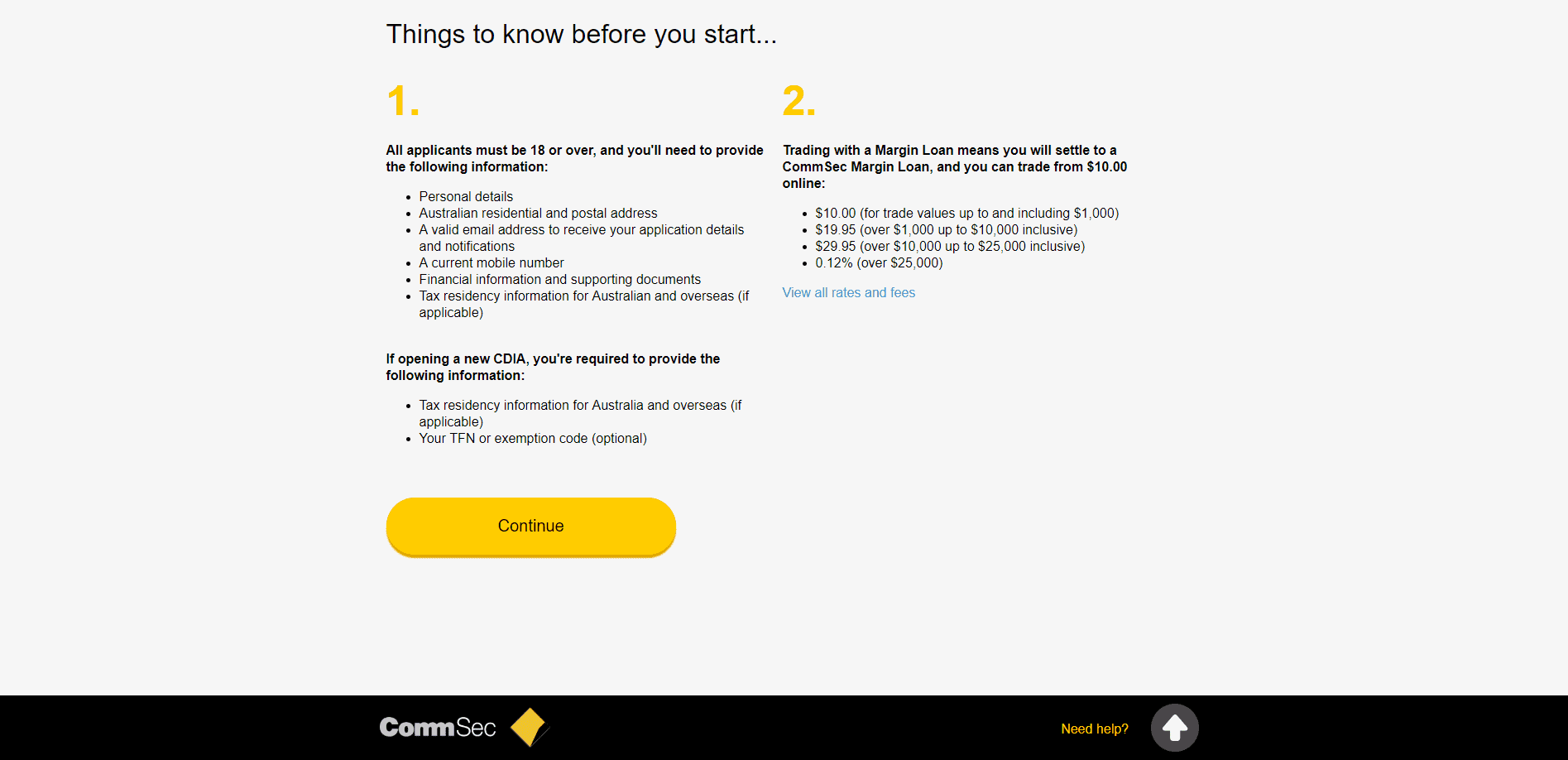A screenshot from a website or app displaying detailed information for prospective applicants. The text at the top reads, "Things to Know Before You Start." The content is divided into two columns. 

The left column lists essential requirements:
1. All applicants must be 18 or over and need to provide the following information:
   - Personal details
   - Australian residential and postal addresses
   - A valid email address to receive application details and notifications
   - A current mobile number
   - Financial information and supporting documents
   - Tax residency information for Australia and overseas, if applicable

Additionally, if opening a new CDIA (Cash Deposit and Investment Account), applicants are required to provide:
   - Tax residency information for Australia and overseas, if applicable
   - Their TFN (Tax File Number) or exemption code (optional)

The right column provides details on trading with a margin loan:
2. Trading with a margin loan means settlements will be to a CommSec margin loan, allowing trades from $10 online. The listed costs for trading are:
   - $10
   - $19.95
   - $29.95
   - 0.12%

At the bottom of the screen, there is a prominent yellow "Continue" button.

Overall, the image effectively outlines the prerequisites and cost structures for new applicants and margin loan trading, guiding users on the necessary steps to proceed.